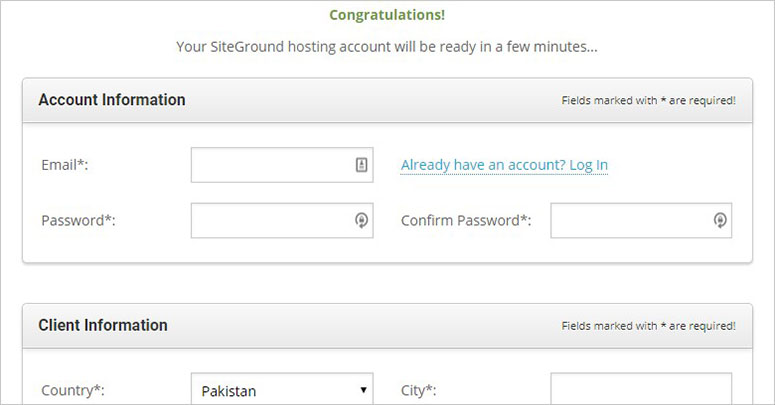The image is a screenshot from the website SiteGround, a web hosting company. The screenshot displays a predominantly white background with green text at the top that reads: "Congratulations! Your SiteGround hosting account will be ready in a few minutes." This message indicates the account registration process for the SiteGround platform. 

The page features several input fields required for account setup. The first section, titled "Account Information," specifies that fields marked with an asterisk are mandatory. It includes an input box for entering an email address, marked by an asterisk. Next to the email input box is a blue link that says, "Already have an account? Log in."

Below the email field, users are prompted to enter a password and confirm it in an adjacent box. Further down is a section for "Client Information," though only part of this section is visible in the screenshot. The visible fields include a dropdown menu to select the country, which currently displays "Pakistan," and a text box for entering the city, which is presently blank like the other input fields.

Overall, the screenshot captures the structured and straightforward account registration process on the SiteGround web hosting platform.